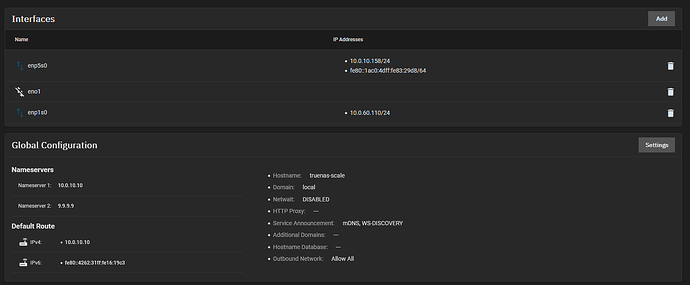The image depicts a user interface for network configuration. On the left side, the interface features a gray rectangle with white text labeled "Global Configuration." Below this title, a section specific to "Name Servers" is visible. It lists "Name Server 1:" followed by an IP address, appearing as "9.9.9.x," and "Name Server 2," also associated with an IP address. Each line of name server information is complemented by a white trash can icon on the right, presumably for deletion actions.

Adjacent to the name server configurations, there's another rectangle, also gray with white text, detailing designed spaces for entering "Name" and "Address" information. This section includes lines for data entry, each aligned with a white trash can icon for removing entries.

In the central part of the interface, several fields are grouped under "Host Name":"Domain" and "Default Route" settings. One of the entries might be associated with a service named "Worker Walt," although the exact position of this detail is ambiguous. The layout seems structured to make network settings management intuitive and straightforward by providing a clean, organized, and easily navigable design.